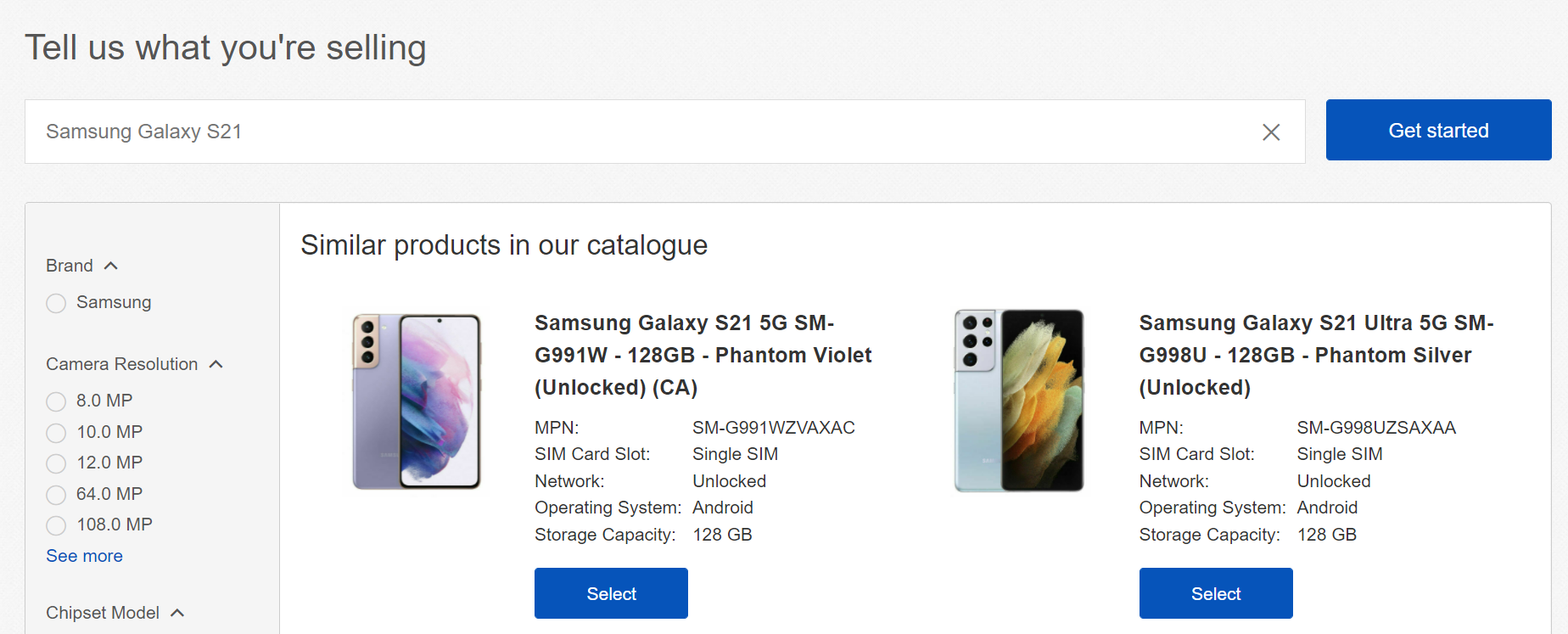Displayed on the webpage is a prompt titled "Tell us what you're selling," leading to a listing for the Samsung Galaxy S21. The page showcases two variants of the phone in distinct colors: Phantom Violet and Phantom Silver. The Phantom Silver version has subtle blue undertones. Both phones feature identical specifications aside from their color differences.

The left sidebar of the page contains filter options, which have not yet been selected. Each phone listing includes a blue "Select" button at the bottom. Shared specifications include an NPN number, a single SIM card slot, network unlock capability, the Android operating system, and a storage capacity of 128 gigabytes.

The main page has a clean, white background with black text, while the filter pane is gray with black text. At the top near the search area, there is a blue "Get Started" button for initiating the selection process.